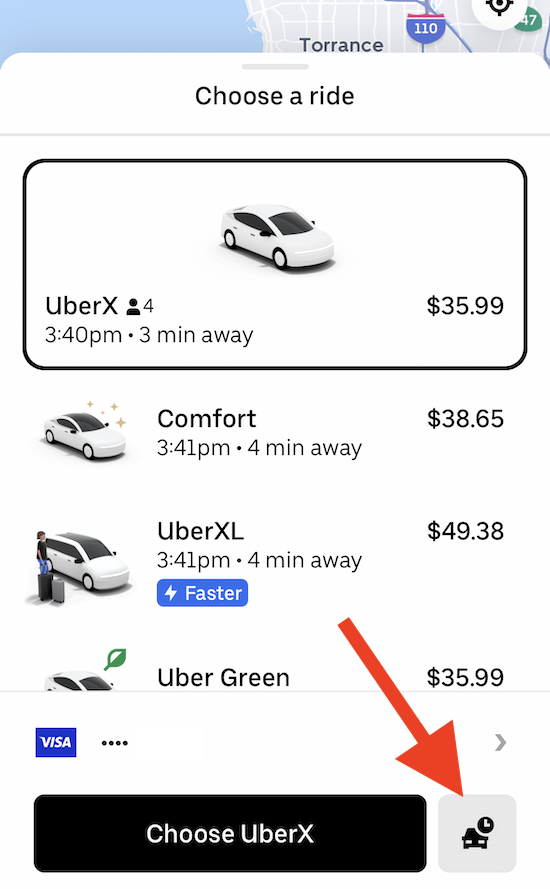The image on the phone screen displays the interface of a ride-hailing app. At the top, a small portion of a map is visible, suggesting the user's current location. Below the map, the screen reads "Choose a Ride," indicating options for different types of Uber services. 

The first option is UberX, shown to be three minutes away with an estimated arrival time of 3:40 PM. This option depicts an icon of a simplistic human figure and a white vehicle, priced at $35.99. 

Following this, the Comfort option is listed with a four-minute arrival, available at 3:41 PM, and priced at $38.65. 

The UberXL service is next, priced at $49.38 and appears to be faster than the previous options.

Another ride option displayed is Uber Green, also priced at $35.99.

In the bottom right corner, there's a clickable gray square highlighted by a red arrow, intending to draw the user's attention to select UberX.